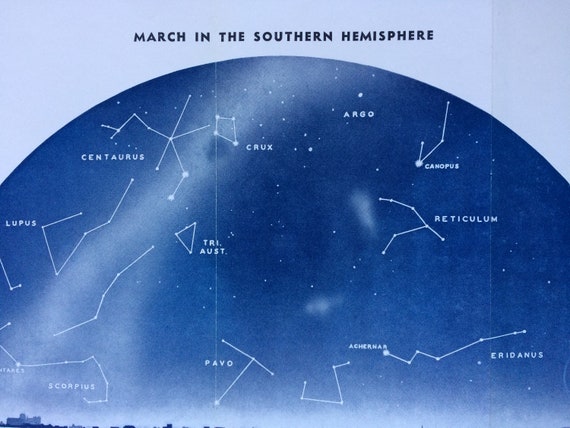This image is a detailed star chart labeled "March in the Southern Hemisphere," depicting various constellations visible during that time of the year. The chart features a blue and light blue background representing the night sky. Within this celestial sphere, numerous stars are depicted as white speckles, with certain stars connected by white lines to outline constellations. Prominent constellations and stars identified on the map include Centaurus, Crux, Argo, Canopus, Reticulum, Triangulum Australe (Triost or Triars), Pavo, Lupus, Scorpius, Eridanus, and several others. The constellations are labeled clearly, providing a comprehensive guide to the Southern Hemisphere's night sky in March.